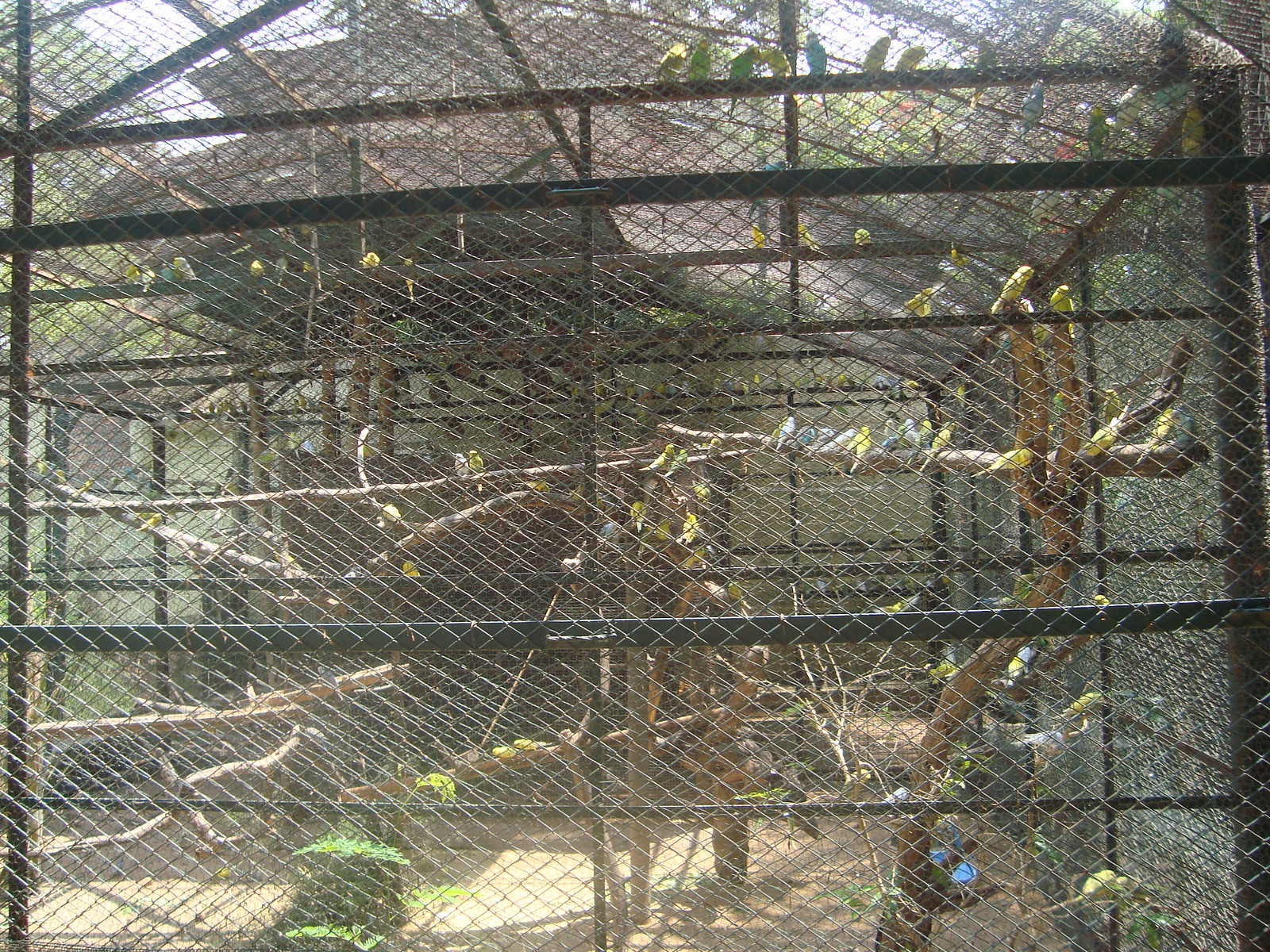This photograph captures a large outdoor aviary on a sunny day. The spacious black-fenced cage, framed with black pipes and a small silver mesh, houses an array of vibrantly colored birds—yellows, greens, and shades of blue—resembling parakeets or small parrots. Tree branches crisscross the interior in various directions, offering perches at different levels, from the lower sections to the very top, where many birds are settled. Some branches host groups of up to a dozen birds sitting close together. At the top of the aviary, the roof consists of the same gated material as the sides, supplemented by a transparent covering for shade. The ground inside is dirt, dotted with green plants and a blue water tray. In the background, a larger structure casts a shadow, suggesting the aviary could be part of a zoo exhibit.